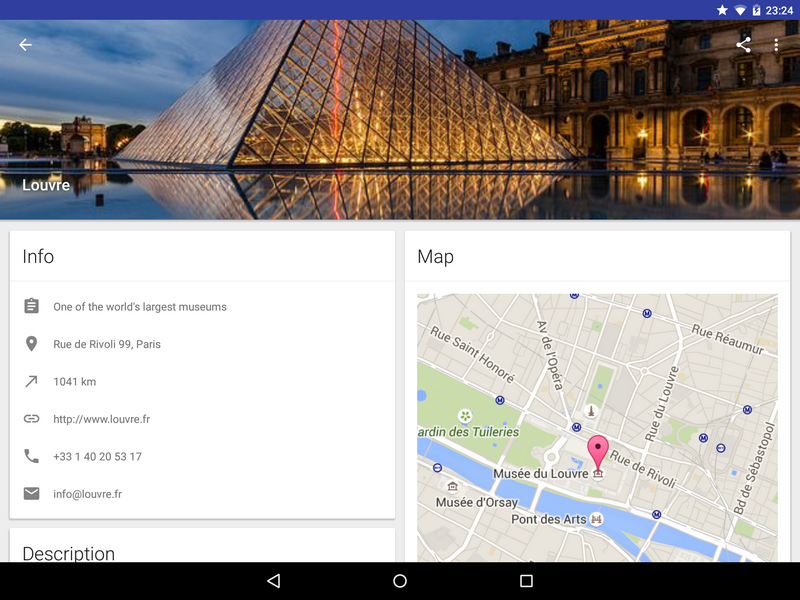The web page features a distinctive and eye-catching design, beginning with a vivid blue banner spanning across the top. Positioned on the far right of the banner is a star icon, next to which a mostly full battery icon and the time reading 23:24 are displayed.

Directly below the banner, the main content is dominated by a striking nighttime photograph of the Louvre. The iconic museum is illuminated, showcasing its grand architectural features against the dark, slightly cloudy night sky. In the foreground, a large glass pyramid, aglow from interior lights, commands attention and adds a modern contrast to the historic backdrop.

On the left side of the image, the word "Info" is prominently featured, followed by vertically arranged light gray text that details key information: "One of the world's largest museums," "Rue de Rivoli 99," "Paris 1041." Below this, there is a link to the Louvre’s official web page, accompanied by a phone number and an email address for further inquiries. 

A white box labeled "Description" appears, though no additional details are provided within this image. To the right of this section is the word "Map" in black text, under which a map of the Louvre's location is displayed, clearly marking the surrounding streets and nearby river.

At the bottom of the screen, a black ribbon with navigation options is visible, including a white back button, a home icon, and a square icon situated to the right. These elements collectively enhance user accessibility and engagement with the webpage.